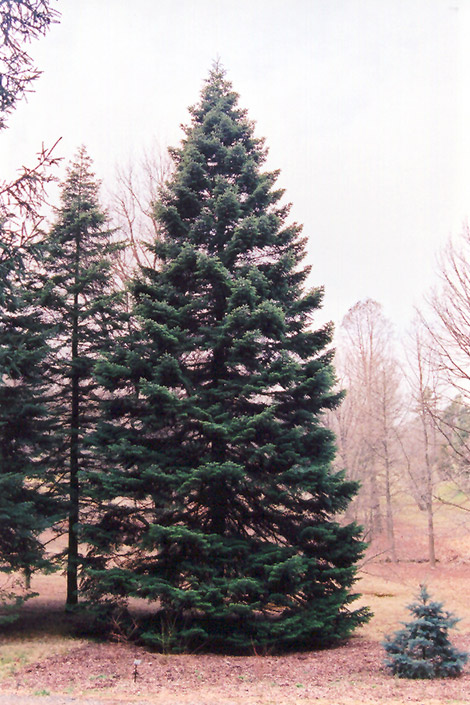The vertically rectangular, full-color photograph portrays an outdoor scene during daytime in what appears to be either fall or early spring, owing to the barren trees devoid of any leaves. The colors are somewhat faded, encompassing hues of brown, light brown, tan, green, dark green, off-white, and a faint yellow. The central focus is a majestic, Christmas tree-like pine tree, standing tall and full in the middle, resembling a tree one might fantasize about placing in Rockefeller Plaza due to its grand stature, likely 20-30 feet tall. To its right, the lower corner showcases a small pine tree amidst some land, and further left, a few scraggly pines dot the side. Surrounding the focal tree, the trees in the background and flanking sides are stripped of leaves, enhancing the sense of cold weather and hinting at the winter season. The sky, occupying the upper right section, is grayish, possibly clouded, accentuating the somber, chill atmosphere of the forested area. This serene landscape, devoid of people, animals, or text, captures the tranquil beauty of nature in its dormant phase.